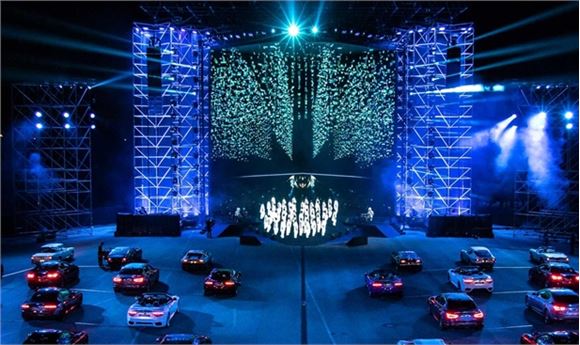The image depicts a digitally rendered outdoor performance venue with a small, flat central stage surrounded by symmetrically arranged parked vehicles, their headlights on, resembling a drive-in show. Tall towers equipped with lights and equipment flank the stage on the left and right, emitting a bright array of stage lights in hues of green, blue, and sparkling white. Above the stage, long strings of hanging lights cascade down, adding to the vibrant atmosphere. The stage hosts what appear to be glowing white figures, though it's difficult to discern whether they are actual people due to the distance and hazy, smoky effects that obscure parts of the scene. The backdrop features glittery and sparkly lights, enhancing the overall luminous and dynamic ambiance of the venue. The vehicles are parked in orderly rows, with their red taillights visible, reinforcing the impression of an audience watching a captivating performance from the comfort of their cars.